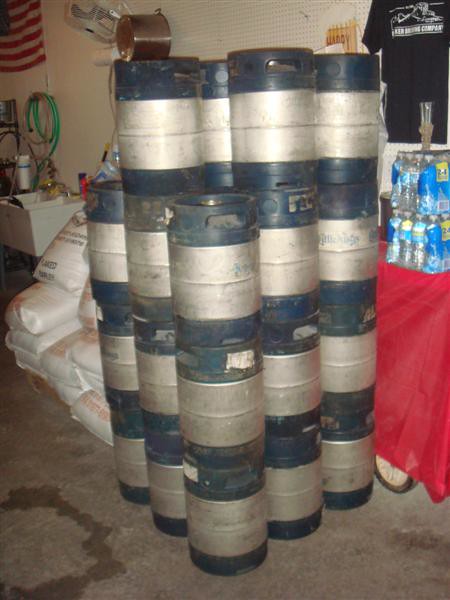This photograph displays an array of beer kegs meticulously stacked atop each other, arranged in a 3x3 grid with an additional loose group of four barrels perched on top, creating a towering structure. Each keg features distinctive dark blue stripes near the top and bottom, with a silver chrome section in the middle, equipped with built-in handles. To the right of the stack, a red tablecloth drapes over a table, supporting two stacks of bottled water, while a blue t-shirt hangs on the wall behind it. The scene is set against a white wall viewed from an angle, and in the background to the left, there is a laundry room sink with a green hose mounted on the wall above it. An American flag is prominently displayed in the top left corner of the image, contributing to the overall setting, which appears to be in a concrete-floored environment.